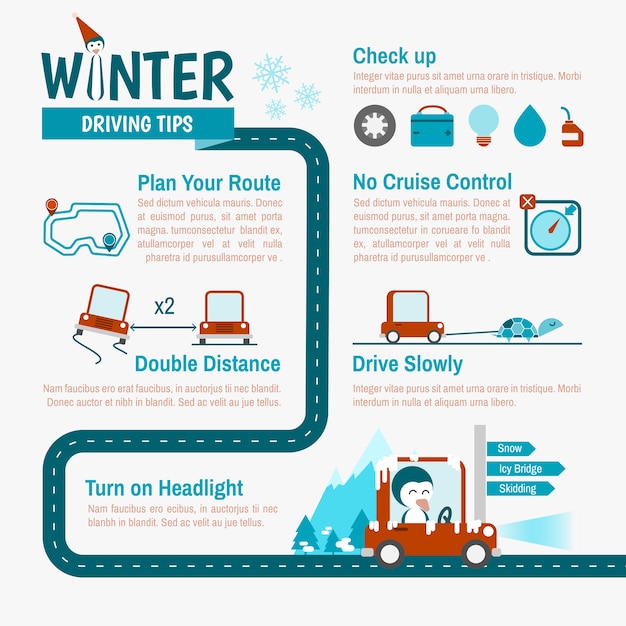The poster, designed in a dark teal and red color scheme with white accents, is an infographic titled "Winter Driving Tips." The letter "I" in "Winter" is creatively depicted as a penguin wearing a tall, conical red hat. The layout of the infographic uses a winding road that guides the viewer through various driving tips. 

Each tip is accompanied by unique graphics and listed as follows:
1. **Plan Your Route** - Illustrated with a diagram of a road map.
2. **Double Distance** - Shown with two red cartoon cars spaced apart to indicate doubling the normal driving distance.
3. **Turn on Headlights** - Depicted by a penguin driving a red car with headlights on, illuminating the road.
4. **Check Up** - Visualized with icons that include a gear, a suitcase, a light bulb, a raindrop, and an oil can, symbolizing a vehicle check-up.
5. **No Cruise Control** - Advised through text without an accompanying image.
6. **Drive Slowly** - Highlighted with a cartoon red car being humorously pulled by a turtle, as well as another image of a penguin driving through snowy conditions with snowflakes falling, and a warning sign that reads "Snow, Icy Bridge, Skidding."

Despite the English titles, the detailed descriptions beneath each tip are written in placeholder text that resembles fake Latin, known as "lorem ipsum." The poster’s overall message is visually engaging and playful, using cartoony elements to emphasize the importance of safe driving practices in winter conditions.